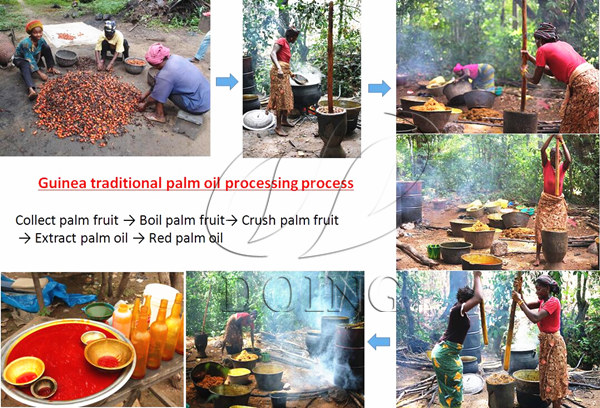This detailed infographic illustrates the traditional palm oil processing process in Guinea, Africa. The central red text prominently states "Guinea Traditional Palm Oil Processing Process," accompanied by the sequential instructions in black text: "Collect palm fruit," "Boil palm fruit," "Crush palm fruit," "Extract palm oil," and "Red palm oil." The infographic features a series of seven photographs on a white background, capturing different stages of this labor-intensive method undertaken by several women.

In the upper left-hand corner, the first photograph showcases three women wearing headscarves, squatting or kneeling around a big pile of orange palm fruit on a mound of dirt in a small clearing within a wooded area. The subsequent photographs provide a step-by-step visual narrative of the process. The second image shows a woman in a long skirt standing over a large black pot, actively stirring the boiling palm fruit. This is followed by an image of another woman using a stick to crush the palm fruit in a big pot.

Further down, the infographic includes an image of a large pot filled with extracted, deep red palm oil, with nearby amber bottles suggesting its eventual storage. The fourth photograph aligns with this, showing a woman leaning over a pot, engaged in the extraction process. Finally, the concluding set of images illustrates two women, one using a stick or pounder in a wooden base to further crush the palm fruit.

Throughout the sequence, the daylight and sunny environment reveal the social and routine nature of this traditional activity, highlighting both the communal effort and the cultural significance of palm oil production in Guinea.